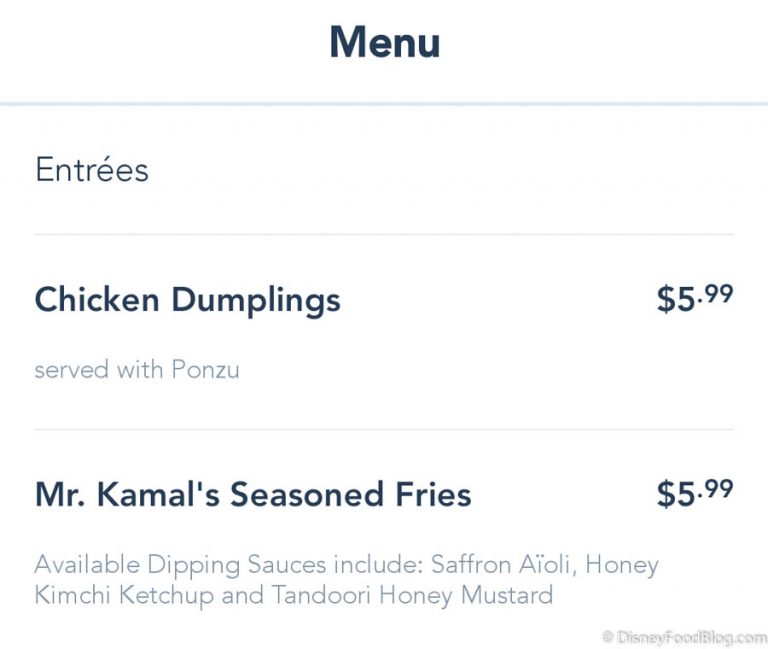The image showcases a menu with "MENU" prominently printed at the top in thick, large black lettering. Below this title, a light blue-gray line horizontally separates the sections of the menu. The section title "ENTREES" is printed in lighter gray text beneath this line. Another line, also light gray but slightly indented from both sides, further separates the content below.

The first item listed is **Chicken Dumplings**, with the name boldly printed and the price, $5.99, alongside. The description "served with ponzu" follows in lighter gray writing. A pinkish-colored fine line separates this item from the next.

The second item on the menu is **Mr. Kammel's Seasoned Fries**, again in bold black letters with the price, $5.99. The description includes "lightly available dipping sauces" such as saffron aioli, honey kimchi ketchup, and tandoori honey mustard, printed in a lighter font. 

On the right side of the menu, there is a watermark or branding mark that reads "DisneyFoodBlog.com".